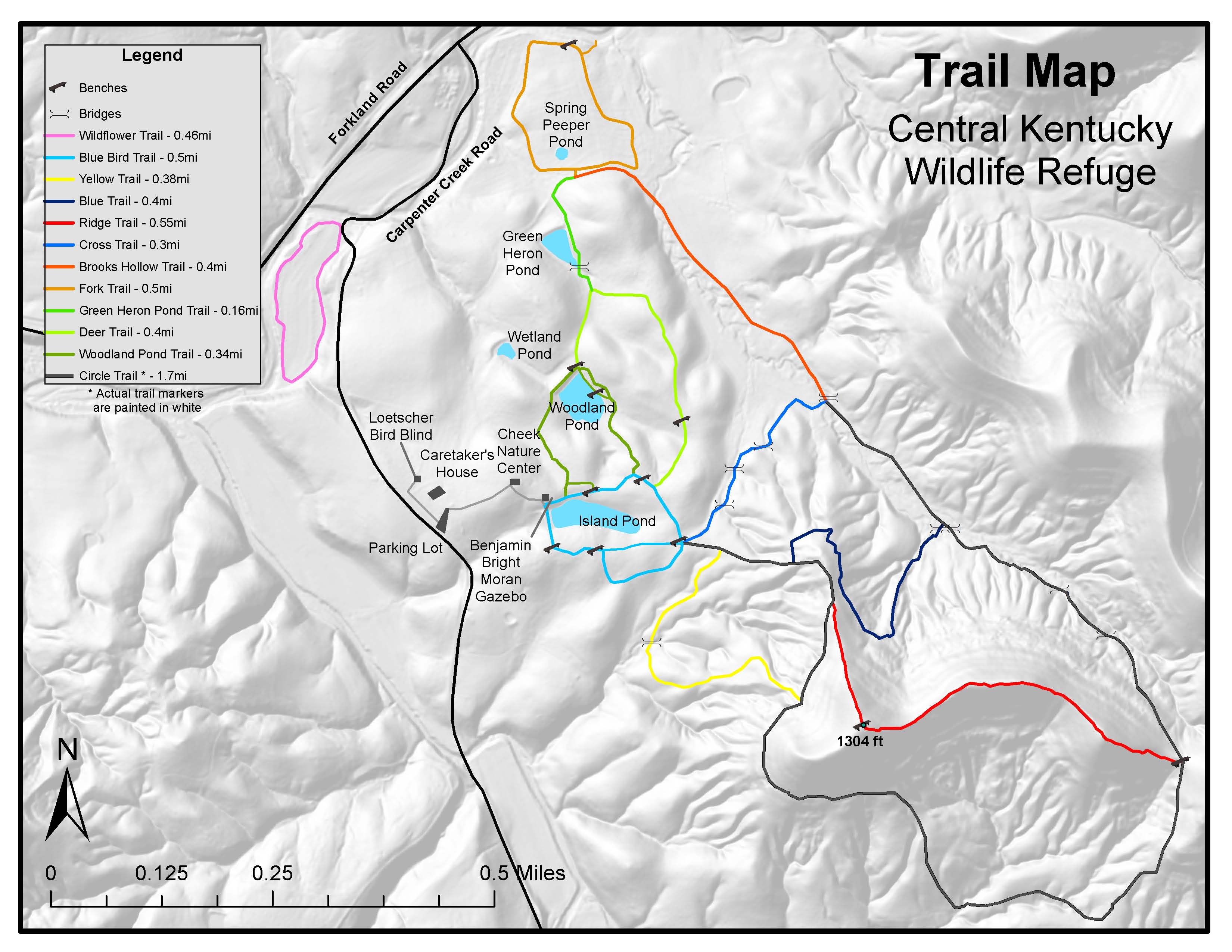This detailed trail map of the Central Kentucky Wildlife Refuge prominently depicts the park's mountainous terrain in a stark white and silver-gray color scheme. The map intricately displays shadows and crevices to clearly indicate peaks and valleys, offering a topographic view of the landscape. The legend, positioned to guide visitors, uses various colors to denote different trails including Bridge, Flower, Bluebird, Yellow, Blue, Ridge, Cross, Brooks Hollow, and Deer trails. Additionally, it highlights key locations such as the parking lot, Benjamin Bright Morin, Gazebo, and the Island Portland, with distances measured to help visitors navigate through the park. Upper-right text reinforces the title: "Trail Map Central Kentucky Wildlife Refuge," making it easy to identify and reference.